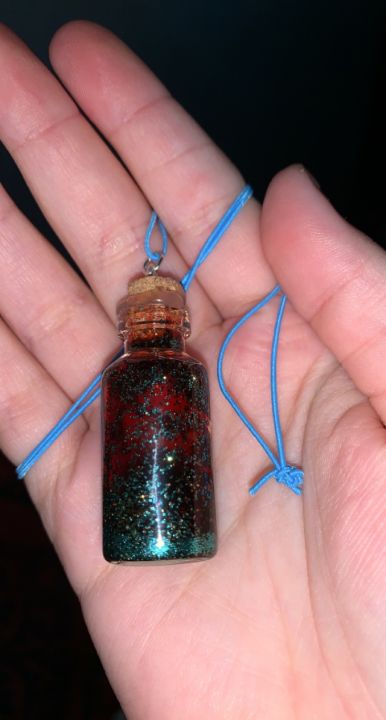In the image, a white person's hand is positioned diagonally, extending from the lower left to the upper right against a completely black background. The lighting is focused on the hand, revealing intricate details. The hand holds a delicate necklace made of a thin, stretchy, light blue string, which is intricately wrapped around four fingers—the thumb, index, middle, and part of the fourth finger. The thumb pinches the end of the string towards the other fingers. Attached to the string, hanging from a small circular metal ring on a cork top, is a tiny glass vial. This vial, possibly plastic, is palm-sized and contains a densely packed dark red liquid resembling hot sauce or nail polish. The liquid has a complex, shimmering appearance with green and black colors intermingled, giving it a sparkly, almost magical quality. The contrast of the black background makes the elements within the bottle and the details of the hand vividly stand out.